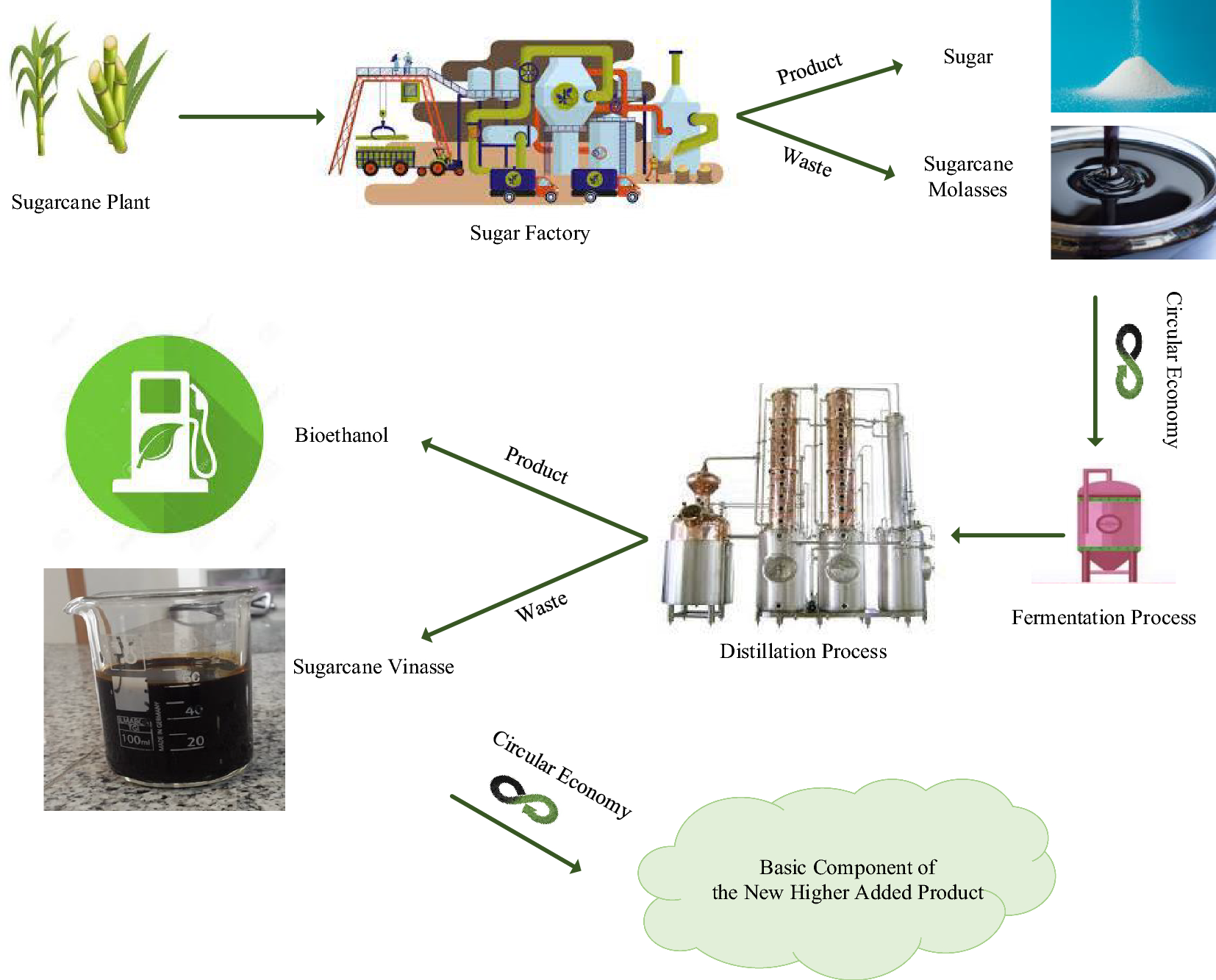The image is a detailed flowchart infographic on a white background illustrating the processing journey of sugarcane plants into various products and their integration into a circular economy. 

In the top left corner, there is a cartoon-like image labeled "sugarcane plant." An arrow points to the right towards a cartoon factory labeled "sugar factory." This factory has two branching arrows: the top arrow labeled "product," leading to an image of white granulated sugar, and the bottom arrow labeled "waste," pointing to a photo of sugarcane molasses.

From the sugarcane molasses, an arrow labeled "circular economy" descends to a pink vat labeled "fermentation process." Another arrow branches left towards the "distillation process," represented by intricate machinery. The distillation process also has two arrows: the top one labeled "product" leading to bioethanol, and the bottom one labeled "waste," pointing to sugarcane vinasse. 

Finally, another arrow labeled "circular economy" arcs downward and to the right, ending in a thought bubble labeled "basic component of the new higher added product." 

This detailed infographic effectively maps out the transformation of sugarcane through various stages, emphasizing the outcomes of each process and their contributions to a sustainable circular economy.